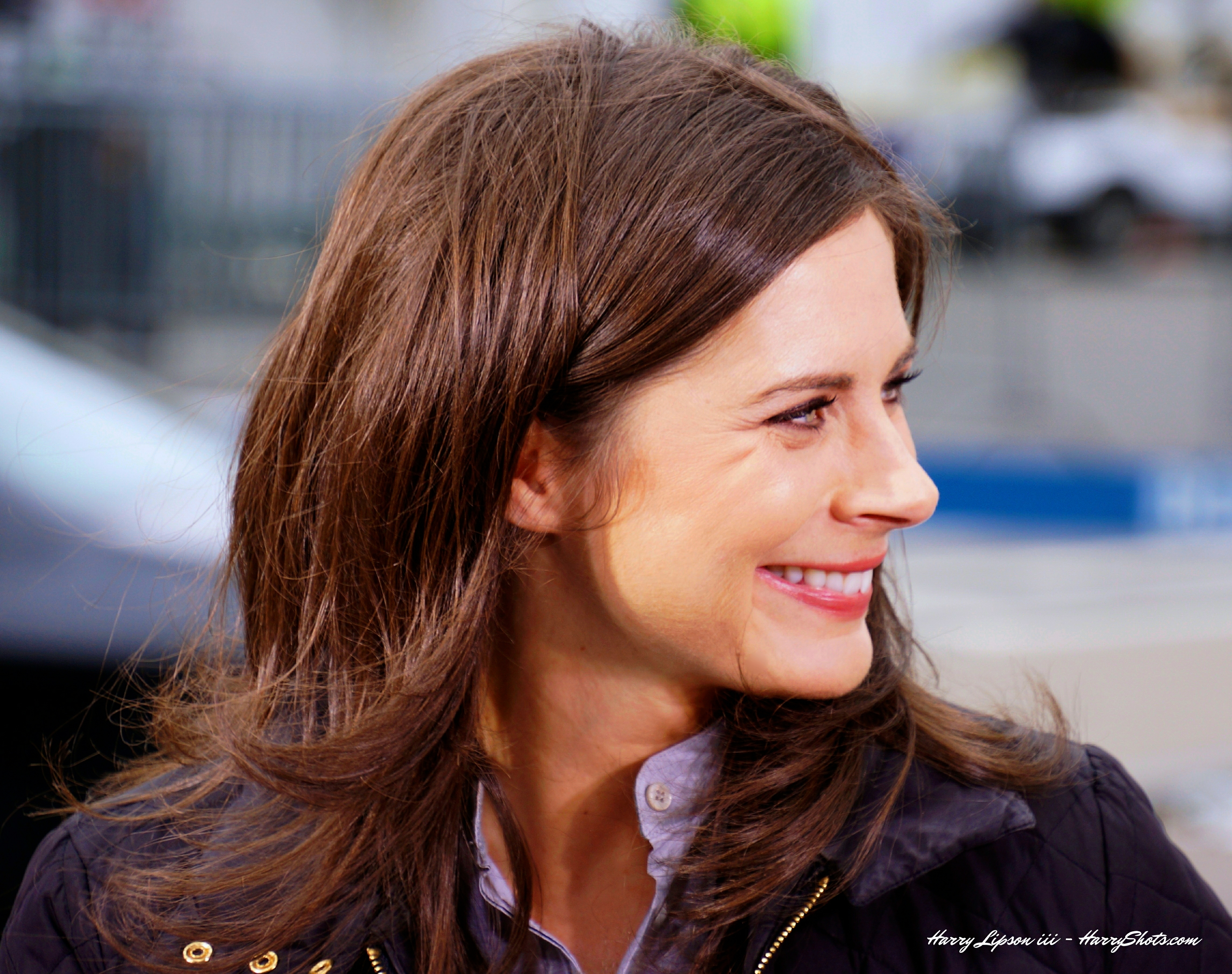This detailed photo features Erin Burnett, who is looking off to the side with a subtle smile, revealing her top row of teeth. She has shoulder-length chestnut brown hair with some strands tucked behind her ear, and light-colored eyes. She is dressed in a dark zip-up jacket over a light blue chambray shirt with visible buttons. The background is out of focus, but discernible elements include the back window of a car, a distant sidewalk with possibly a parking area, a sign, a bit of a fence towards the upper left, and various colors such as white, blue, light brown, and green above her head. The bottom right corner of the image is marked with "Harry Lipson III-HarryHarryshots.com."